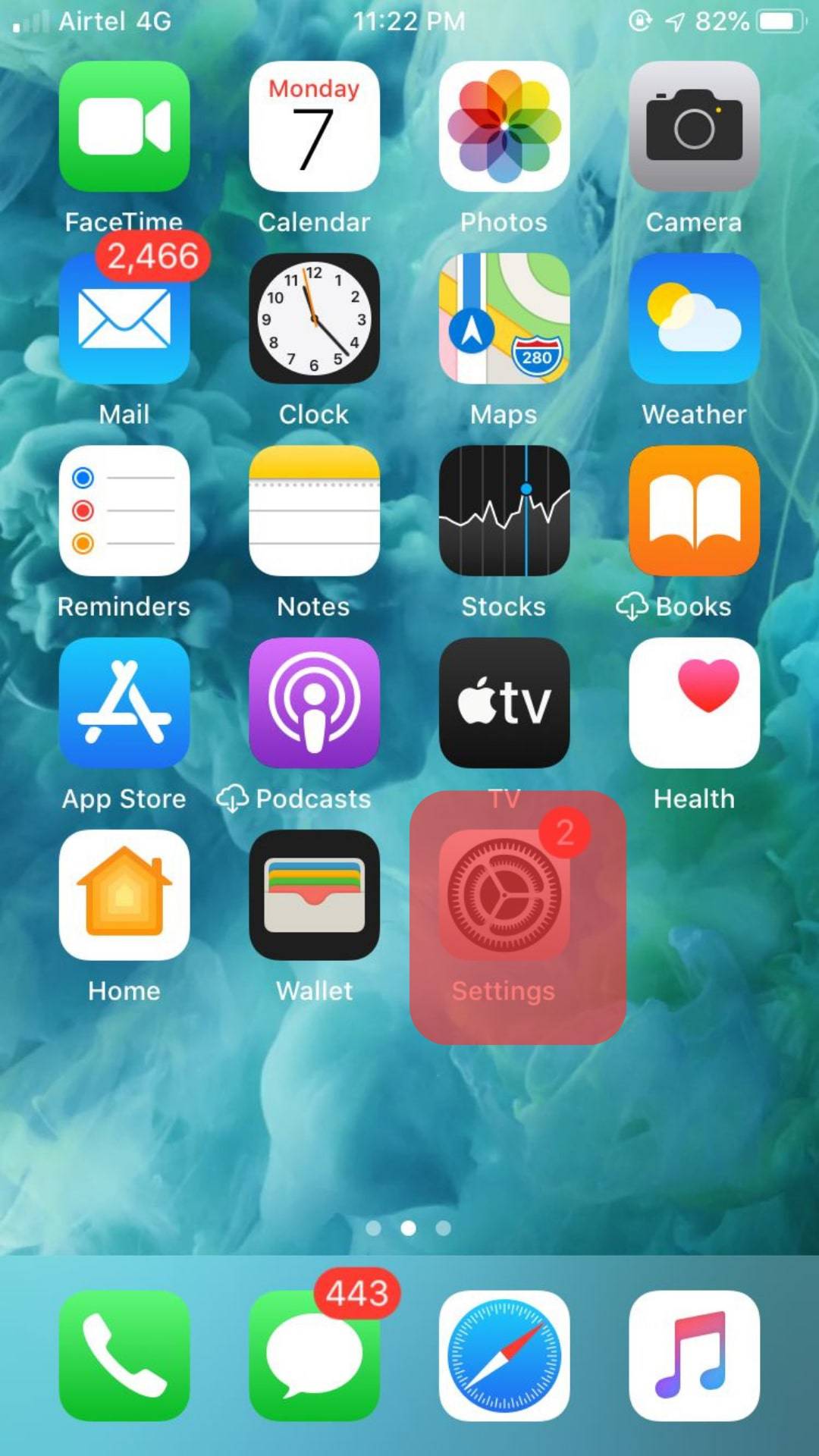The phone screen displays various details at the top, including the "Airtel 4G" network with one signal bar, the time "11:22 p.m.", an 82% battery level, and numerous app icons. Specifically, there are 19 different icons arranged in four rows of four, with three icons alone at the bottom. The wallpaper is a turquoise color resembling smoke. 

At the top left corner of the screen, there is a green box labeled "FaceTime" with a camera icon. To its right, a white box marked "Calendar" shows the date as "Monday 7." Next is the "Photos" icon, followed by a light purple box named "Camera." There’s also a blue box labeled "Mail," which shows 2466 notifications. 

Onwards, a black box with a white clock icon signifies the "Clock" app. Finally, the app to the right of this one displays the "Maps" icon, completing the detailed arrangement of apps on this turquoise smoke-themed background.